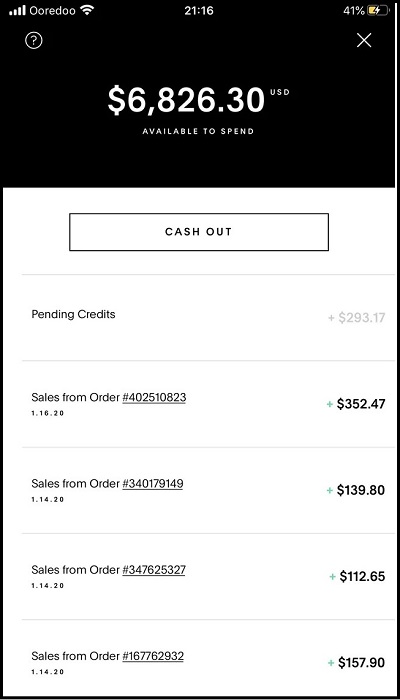The image is a detailed screenshot of a cell phone display showing financial information. At the top, on a black background with white text, several status icons are visible: a full four-bar signal strength symbol indicating maximum data speed or power, the network name “Ooredoo,” and a full-strength Wi-Fi signal. The time is displayed as 21:16, and the battery percentage on the far right shows 41%.

Directly below the status bar, also on the black background, there is a prominent piece of financial information stating "$6,826.30 USD available to spend."

The rest of the information is displayed on a white background. A tab labeled "Cash Out" is prominently visible. Below this, the text "Pending Credits" shows a value of $293.17.

Next, detailed sales information from three different orders is listed, each underlined and accompanied by green plus signs next to the amounts:

- Sales from order number 402510823: $352.47
- Sales from order number 347625327: $112.65
- Sales from order number 167762932: $157.90

Each of these sales entries is followed by the date "1.14.20."

There are no additional identifiers or personal information included in the image.